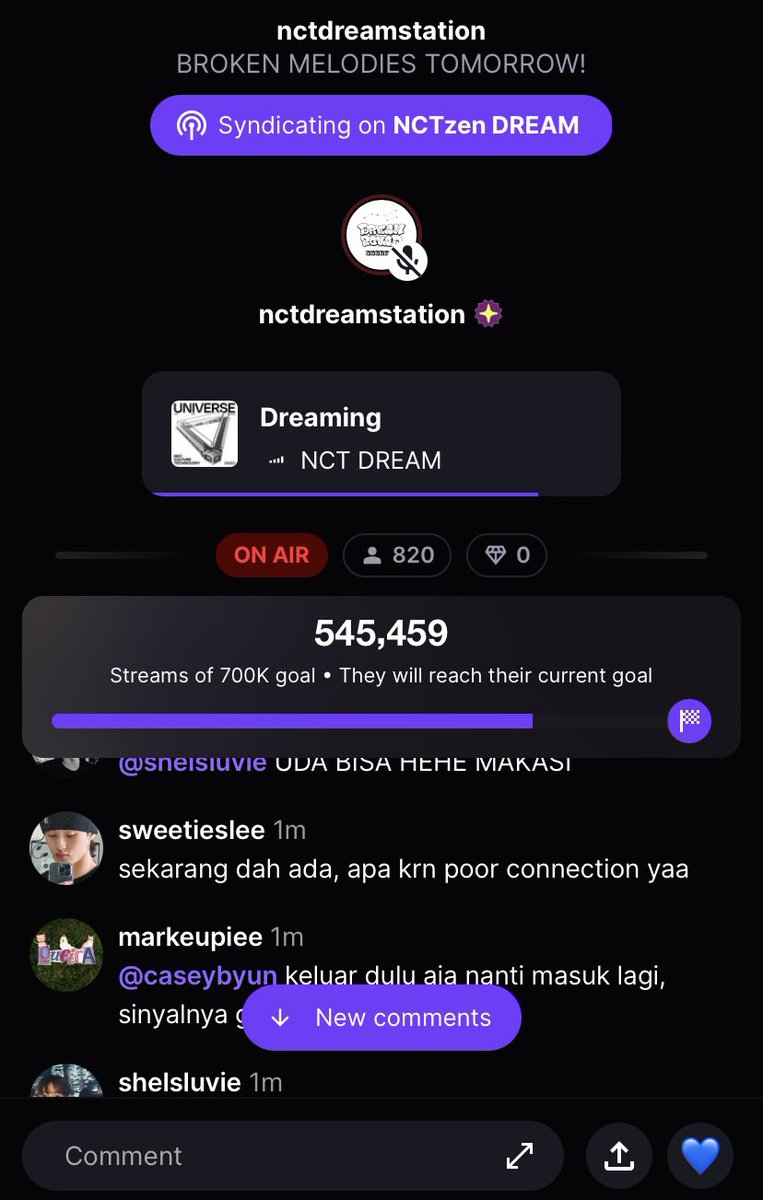The web page appears to be a music streaming service, specifically featuring NCT Dream Station. At the top, there is a black header with the title "NCT Dream Station" in white letters and the text "Broken Melodies Tomorrow." Below this, there is a button labeled "Syndicating on NCT Zen Dream." Another button, which seems to have a microphone icon that is struck out, suggests that the microphone is turned off.

Further down, there's another black rectangle containing an image of a triangle, which resembles a harp. This section is labeled "Dreaming" with "NCT Dream" written underneath. A prominent red button is lit up with the text "On Air," indicating that the broadcast is live, and it shows "820 watchers or subscribers." The stream has achieved 700,000 streams towards a goal. The current goal count is listed as 545,459.

The section also displays the tracks being played and includes a feature that allows users to comment.